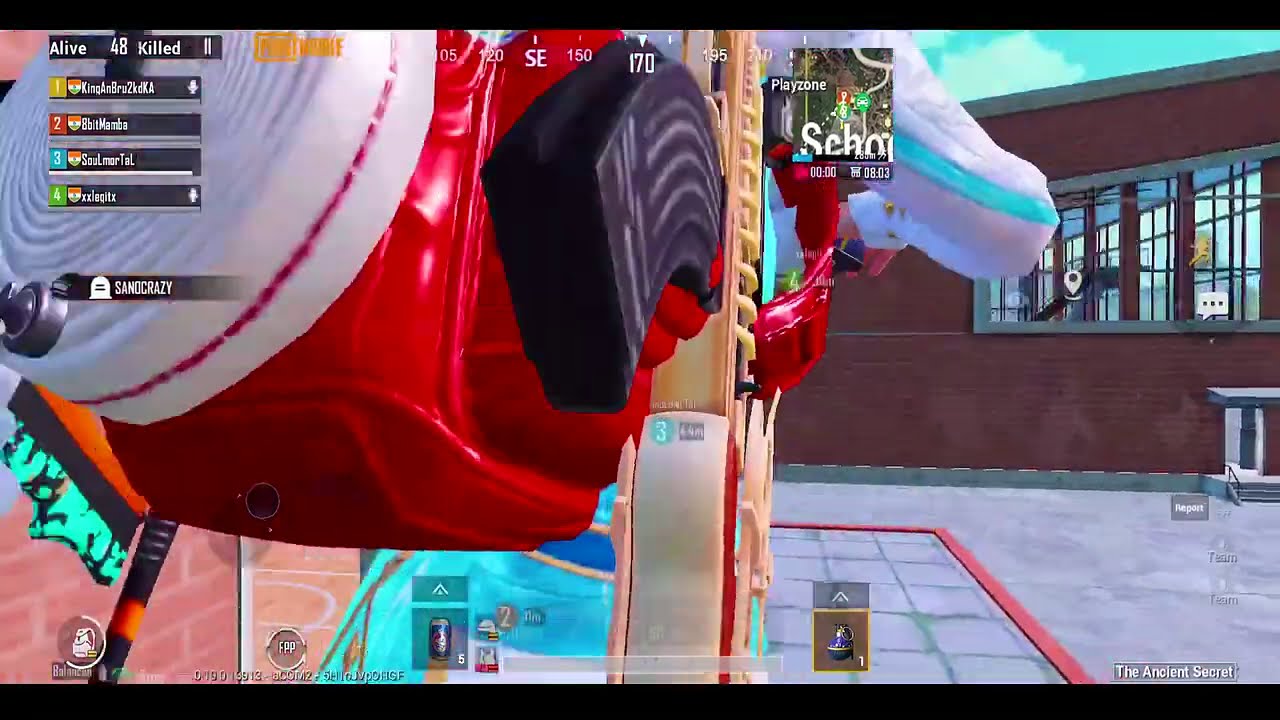The image is a detailed screen grab from a colorful video game, likely Fortnite or PlayerUnknown's Battlegrounds, captured from a high angle. The most prominent feature is a character in the foreground wearing a white jumpsuit with blue accents along the rims. She has a thick red backpack dominating the center of the frame, with a rifle slung over her shoulder. The floor below is a mix of concrete and purple hues, while a red brick building with a visible window dominates the background. A vertical beige structure with various colors and items, including something black, purple, and blue, stands in the middle of the scene. The image also shows turquoise, peach, and mauve colors on the lower left side. The game's user interface displays various indicators: a live counter at the top showing 48 alive and 11 killed, a compass meter, and icons for grenades and energy drinks at the bottom. The player appears to be part of a four-person party.